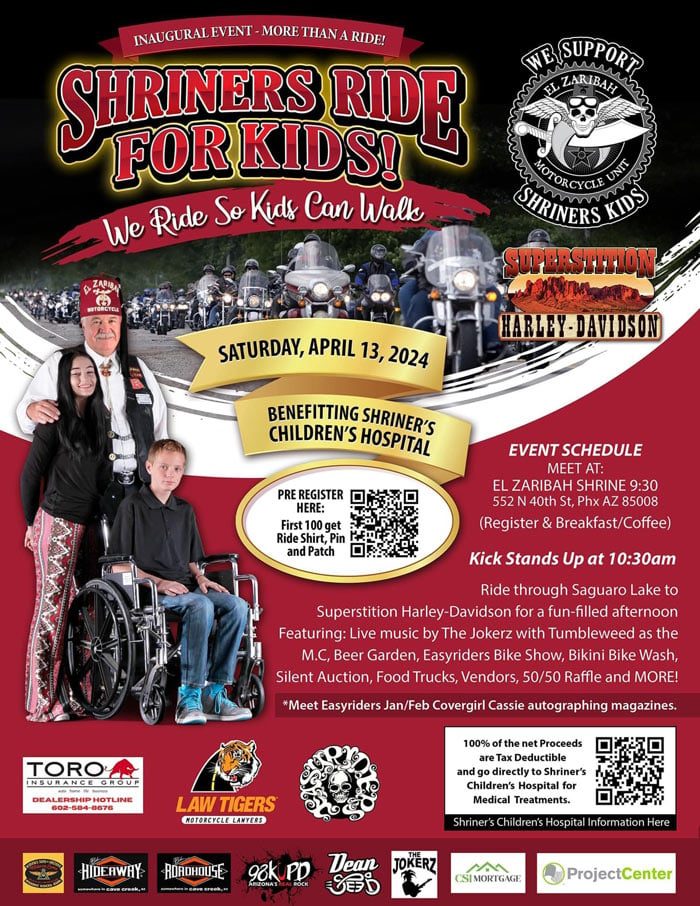This detailed poster for the inaugural Shriners Ride for Kids event prominently features the title in striking red letters at the top, "Shriners Ride for Kids: More Than a Ride - We Ride So Kids Can Walk." Central to the poster is a vivid photograph depicting a long string of Harley-Davidson motorcycles, illustrating the main event, a motorcycle ride. Towards the middle, essential event details are laid out, including a placard with the event's date, Saturday, April 13th, 2024, and a registration QR code, accompanied by information that informs attendees about its purpose of benefiting Shriners Children's Hospital.

To the left of this central information, a touching image displays an older gentleman in a traditional Shriners hat, donning a white button-up shirt and black vest. He stands warmly beside a young girl and a boy in a wheelchair, who appears visibly somber. This photograph underscores the event's heartfelt mission. On the right-hand side, the event schedule is detailed for participants.

At the bottom of the poster, white letters on a red background communicate the day's agenda. This section is complemented by a dozen small advertisements, each featuring logos of the sponsoring organizations that support this charitable cause. The overall aesthetic is dominated by red and gold hues, enhancing the poster's festive yet earnest appeal.